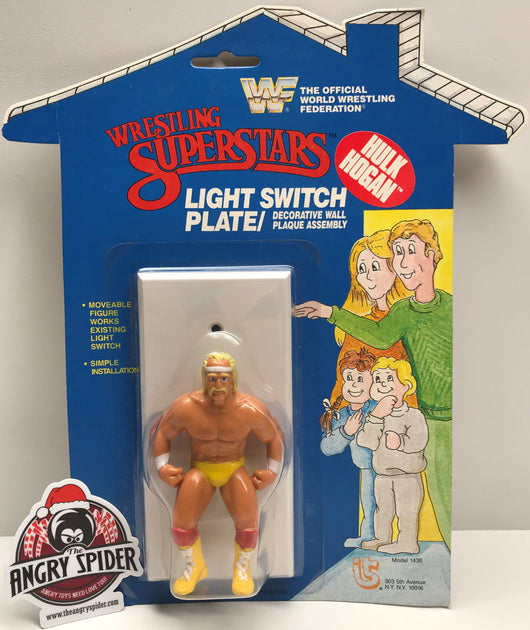The image depicts a whimsical Hulk Hogan light switch plate in its original packaging, designed to bring a humorous twist to a functional household item. The packaging itself is charmingly shaped like a blue house with a white shingled roof and a small chimney, adorned with various labels and text. Prominently displayed within a white, door-shaped rectangle at the center is a small plastic figure of Hulk Hogan, standing in a characteristic wrestling pose with slightly bent knees, arms at his sides, and fists clenched. He wears his iconic yellow shorts, white wristbands, white boots with red toppers, and a yellow headband, complete with his signature blonde hair and mustache.

At the top of the house-shaped packaging in bold red letters, it prominently reads "Wrestling Superstars," with “The Official World Wrestling Federation” logo positioned above. Additionally, a red oval label angled at a 45-degree angle features "Hulk Hogan" in large white letters. To the right side of the packaging, there is a cartoon family of four, dressed casually, visually engaging with the light switch: a blonde man in green attire, a woman with long blonde hair, and two children in light gray and blue outfits, all smiling and appearing delighted by the novelty item.

In the bottom left corner, the branding reveals an "Angry Spider" logo, depicted as a festive creature with a Santa hat, hinting at the manufacturer of this amusing product. Overall, the image blends practical utility with playful nostalgia, showcasing a decorative wall plaque assembly sure to entertain wrestling fans and bring a unique touch to any space.